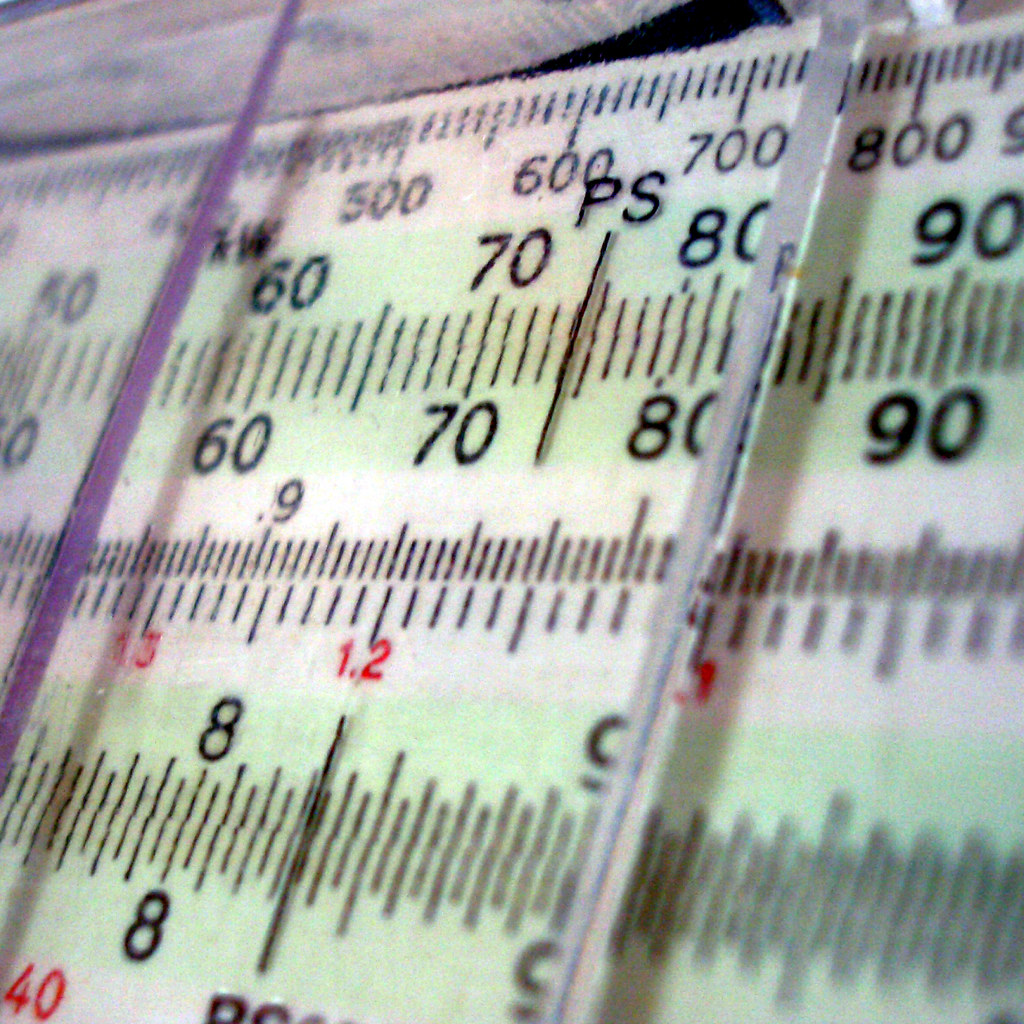This square image presents a detailed close-up of the face of a measurement device, specifically focusing on a gauge that measures an unspecified unit, presumably PS. The gauge features two scales, aligned one above the other. The entire readout, including the range indicators, is rotated approximately 30 degrees clockwise. The scale on the left side is highlighted with a purple bar and a black line, while the right side features a metallic aluminum bar. Both scales are predominantly white with green center bars. The visible numerical range on the scales spans from 60 to 80 PS on the upper scale, and from 7.5 to 9 on the lower scale, though the latter is partially cropped and thus not fully legible.